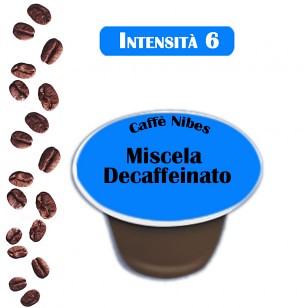This illustration features a detailed product image of a coffee pod set against a white background. Dominating the top section of the image is a blue rectangle with white capital letters reading "INTENSITA 6," indicating a medium-strength coffee. Below, the central focus is the coffee pod itself, resembling a Nescafé pod, with a blue circle on the lid inscribed with "Café Nibes." Prominently across the center of the blue lid, in larger brown letters, is "Miscela Decaffeinato." The pod's body is brown, complementing the imagery. Additionally, a cascade of dark brown coffee beans is arranged along the left border, adding depth and context to the product's depiction.